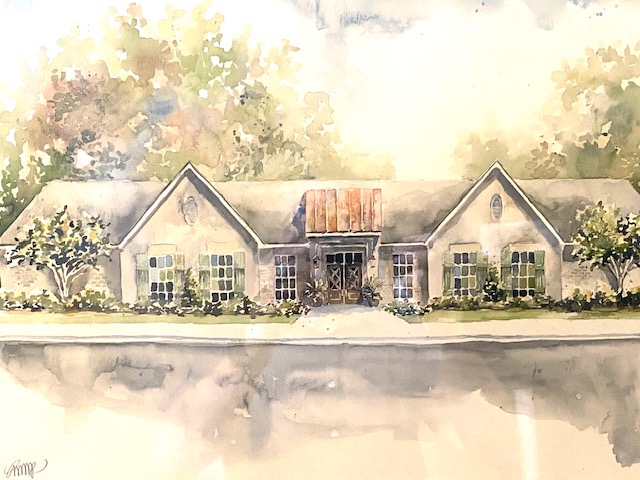This detailed watercolor painting depicts a symmetrically designed house with a distinctive front facade featuring two pointed sections and a prominent, brown door at its center. The house is adorned with numerous window panes along its sides, each with varying colors that add a unique touch to the structure. In front of the house lies what appears to be a pool or shallow body of water, evidenced by the reflection of the house, though the water itself is rendered in soft gray, cream, and pastel hues rather than blue. 

A neat, green garden with vibrant plants and a tree on either side frames the foreground, while tall, lush trees stand majestically in the background. Sunlight filters through, illuminating the scene with bright and airy colors that suggest a sunny day. The color palette throughout the painting includes delicate light purples, pinks, and yellows, giving it a warm and inviting atmosphere. 

At the bottom left corner, the artist's illegible signature subtly marks the piece. The overall effect is a harmonious blend of nature and architecture, captured in delicate, light, and slightly splattered watercolor strokes.